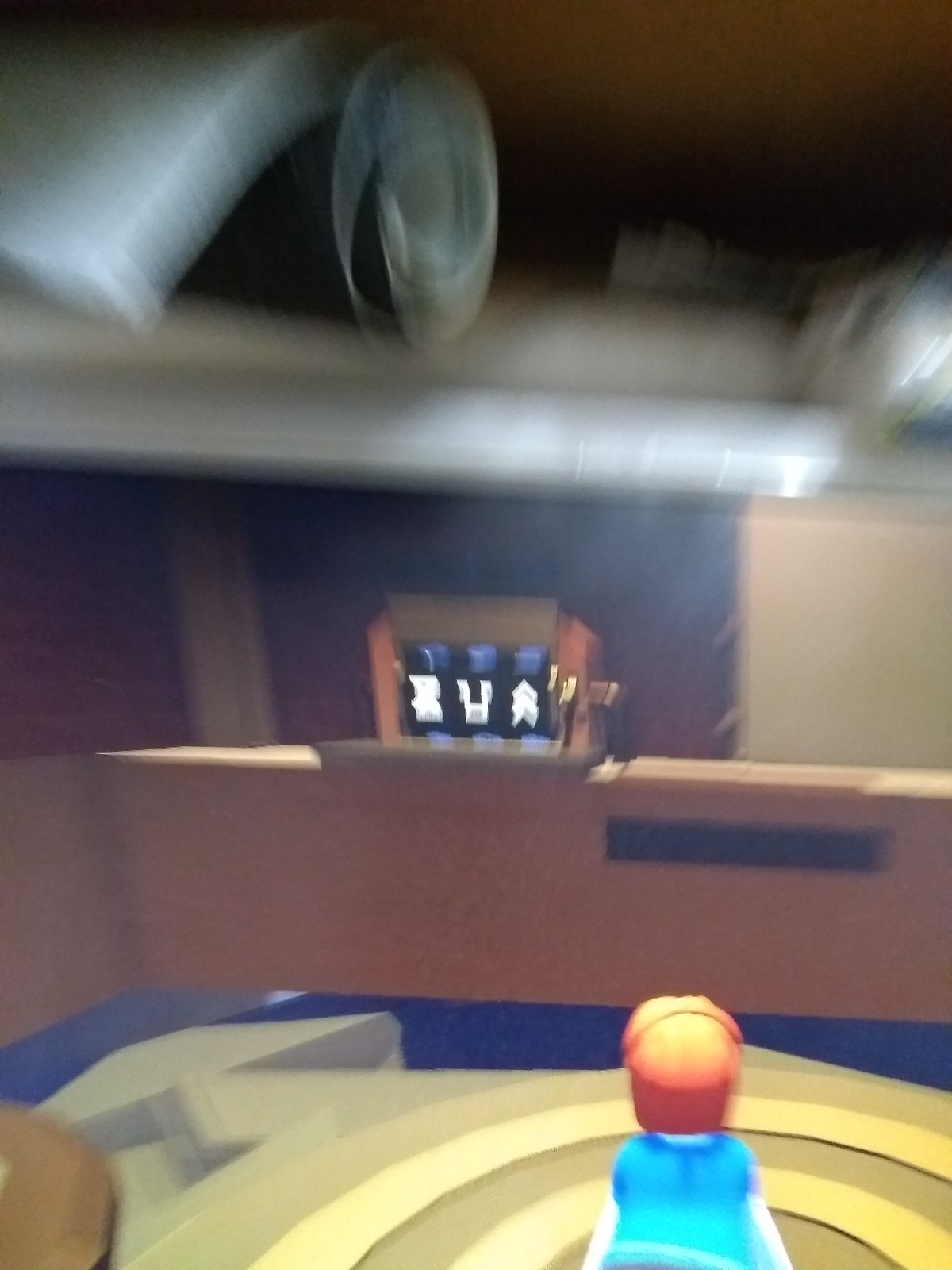This slightly blurry image appears to depict a scene that might be from a computer game, characterized by subpar graphics. In the bottom portion of the photo, a figure resembling a Lego character is visible, viewed from behind. The Lego-like figure sports light brown to gingery hair, transitioning to a darker brown at the bottom and is styled to shoulder length. The character is dressed in a blue top with white sleeves. 

The setting features an abstract, patterned floor, adding to the whimsical atmosphere. In the foreground, a brown counter resembling those found in Chinese takeaway restaurants is prominent, complete with a black kick plate at its base. Above this counter, there is a lit-up box with illuminated and slightly blurred letters that read "ZUA." The backdrop consists of large brown pieces of material mounted on the walls, further enriching the scene with textured, earthy tones.